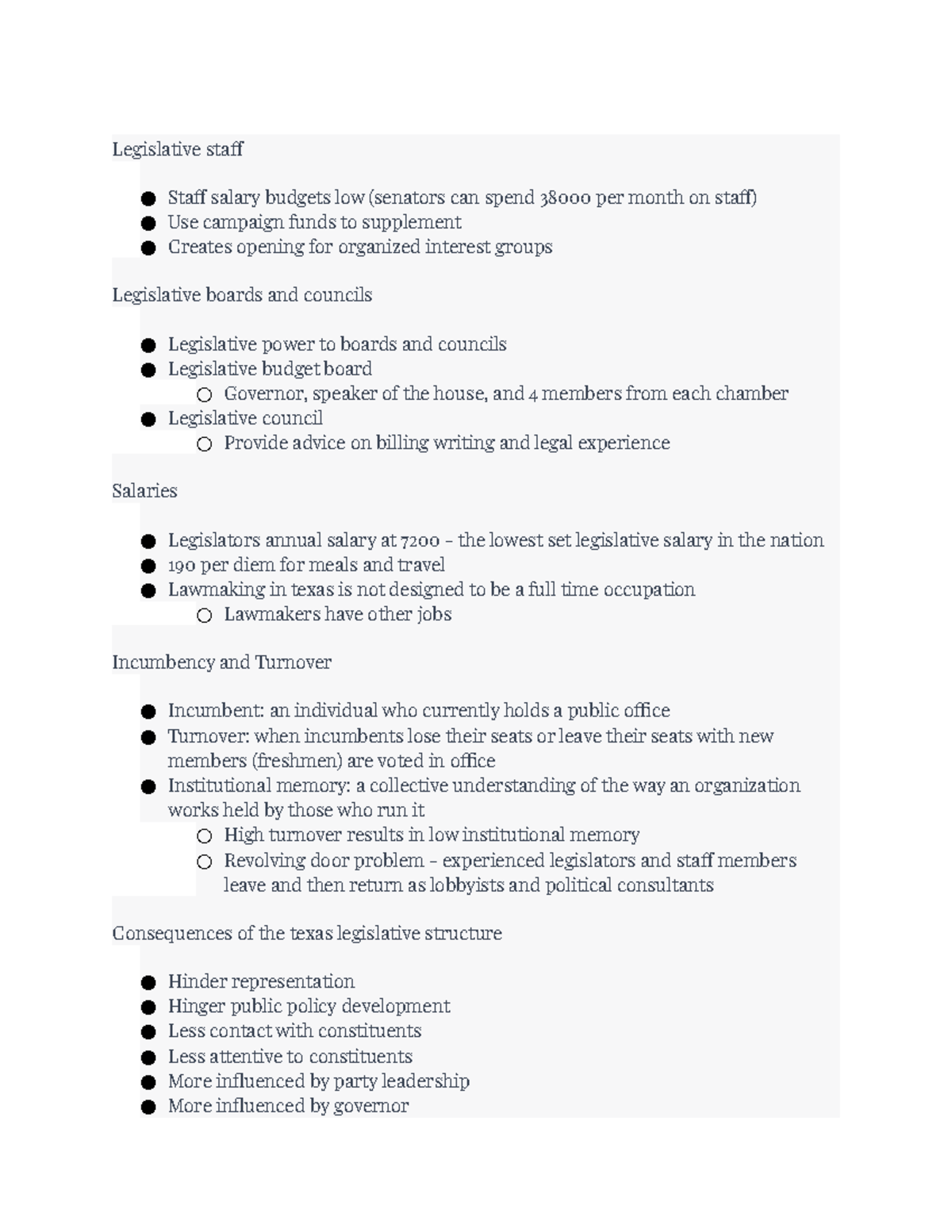"**Detailed Guide on the Structure and Challenges of the Texas Legislature**

This infographic presents a comprehensive overview of the various components and issues within the Texas legislative system, set against a gray background.

**Staff Salary Budgets:**
- Senators in Texas have a monthly staff salary budget of $38,000.
- Legislators can use campaign funds to supplement these salaries, potentially opening avenues for organized interest groups to exert influence.

**Legislative Boards and Councils:**
- Legislative power is delineated to specific boards and councils.
- The *Legislative Budget Board* includes the governor, the speaker of the house, and selected members from each legislative chamber.
- The *Legislative Council* provides essential advice on bill writing and offers legal expertise.

**Salaries:**
- Texas legislators have an annual salary of $7,200, the lowest legislative salary in the nation.
- They receive a $190 per diem for meals and travel, reflecting that lawmaking in Texas is not intended as a full-time occupation, similar to many other states.
- Consequently, many lawmakers hold additional jobs outside the legislature.

**Incumbency and Turnover:**
- An incumbent is a current officeholder, while turnover refers to the replacement of incumbents who lose their seats.
- High turnover rates result in a loss of institutional memory, the collective insight on the workings of the organization, which can prove detrimental.
- The revolving door problem, where officials frequently cycle in and out, exacerbates issues of continuity and institutional knowledge.

**Consequences of Texas Legislative Structure:**
- The structure hinders effective representation and the development of public policy.
- Lawmakers have reduced contact and are less attentive to constituents due to other job commitments, making them more influenced by party leadership and the governor.

Overall, the infographic highlights several key challenges faced by the Texas legislature, likely intended as notes for an educational setting."